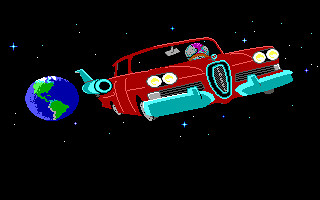This image is a small, retro-styled, pixel art illustration reminiscent of an older video game. The rectangular frame captures a night-time space scene with a black sky dotted with stars. Toward the left of the image, the planet Earth is depicted with recognizable green landmasses and blue oceans, illuminated on one side as if the sun is shining from the left. Central to the image is a red, classic 1940's American car, akin to an Edsel, complete with large chrome front grills, a big emblem on the front, and double yellow headlights. The car also has a rocket-type propeller near the rear fender, hinting at its unconventional ability to float through space. Although there's a figure behind the wheel, their features are indistinct; the head appears round and blue with a hint of pink on top, suggesting either a headdress or some other unique detail. The car moves away from Earth, adding a sense of adventure to the scene.